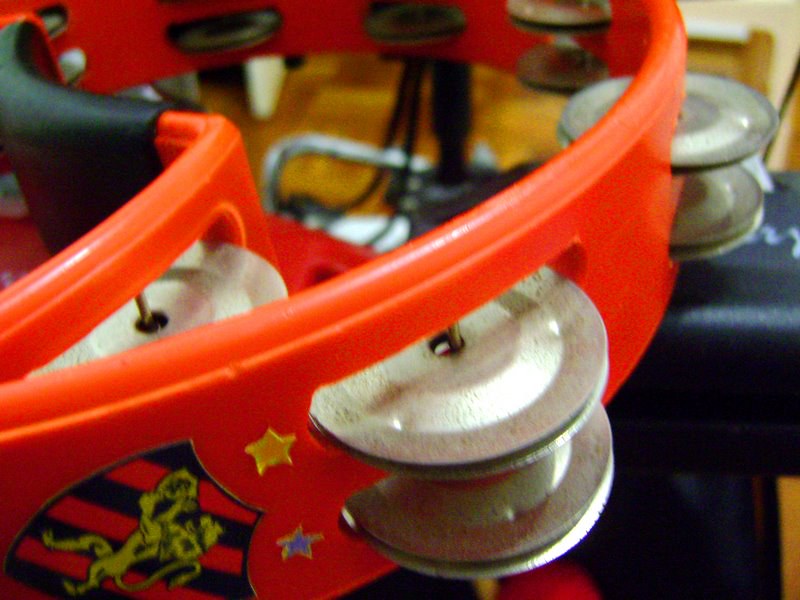This is a close-up photograph of a comma-shaped orange tambourine, often used in schools. The tambourine features a black handle for comfortable playing. On the tambourine's surface, there are two slightly peeling stickers: a blue star and a yellow star, along with a heraldic emblem displaying a black and red shield with a yellow lion standing on its hind legs. The tambourine includes two pairs of silver metal discs positioned on either end. The background reveals a lightly scratched, light brown wooden floor, partially obscured by what appears to be a black chair arm and some metal bars and black cables, possibly components of a music stand or a drum kit.